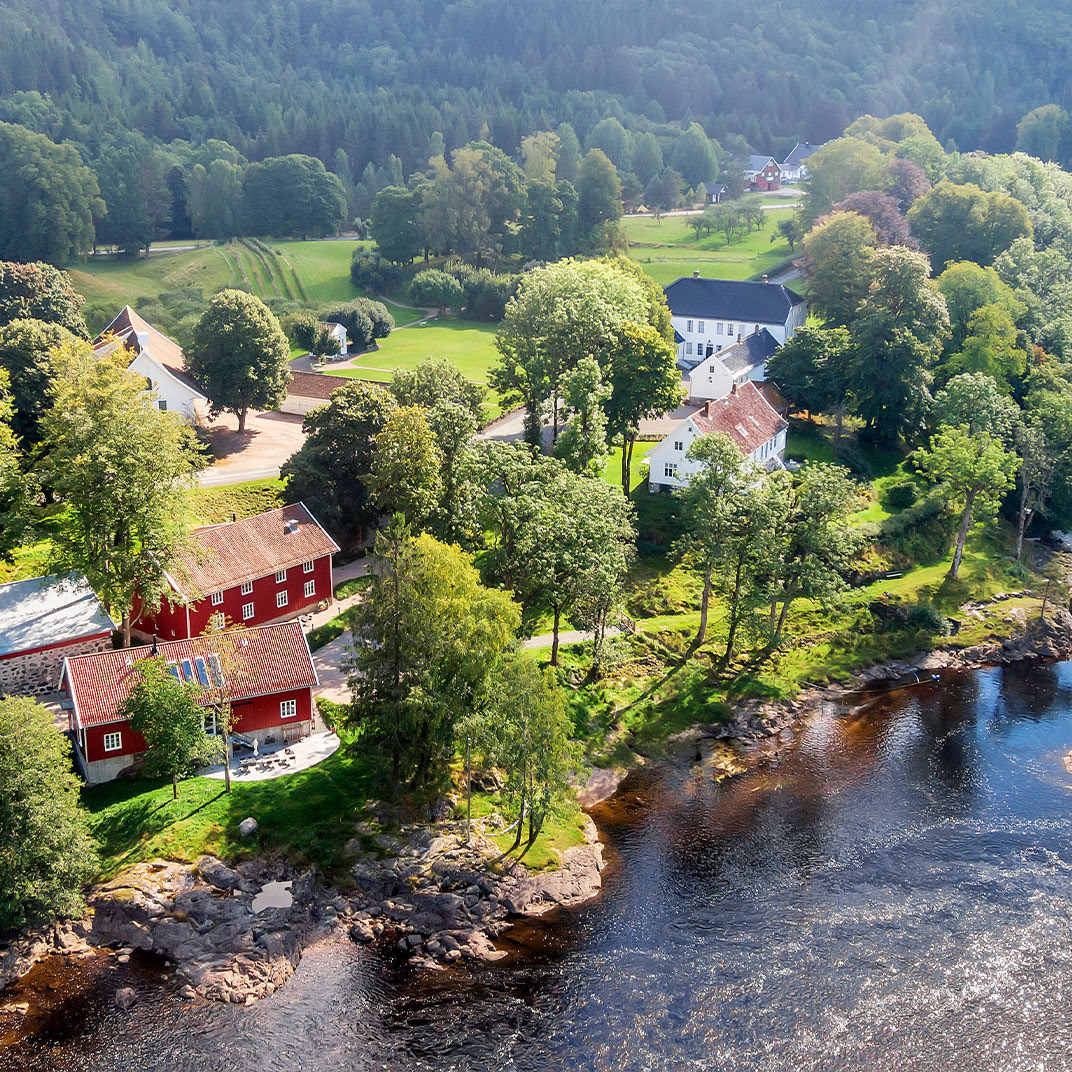This aerial image captures a serene, picturesque village nestled beside a clear yet dark-colored river. The water, revealing glimpses of algae and shadows, seems to be in gentle motion with subtle breaks suggesting mild rapids. The riverbank is adorned with vibrant greenery and meticulously manicured lawns. Prominent in the village are several houses, including two red ones with orangish-red roofs which could be related, possibly one serving as a guest house. Additional dwellings include a dark blue-roofed white house, another orangish-red roofed white house, and an off-white house with a brown roof. Cement paths meander through the village, enriching the idyllic scene. Large, well-tended trees proliferate around the houses and stretch into the background, where a dense, darker forest lies under diffused sunlight, adding to the tranquil atmosphere. The village, possibly reminiscent of a Scandinavian locality like Norway or Finland, appears thoughtfully planned and spaciously arranged, enhancing its charm and inviting serenity.